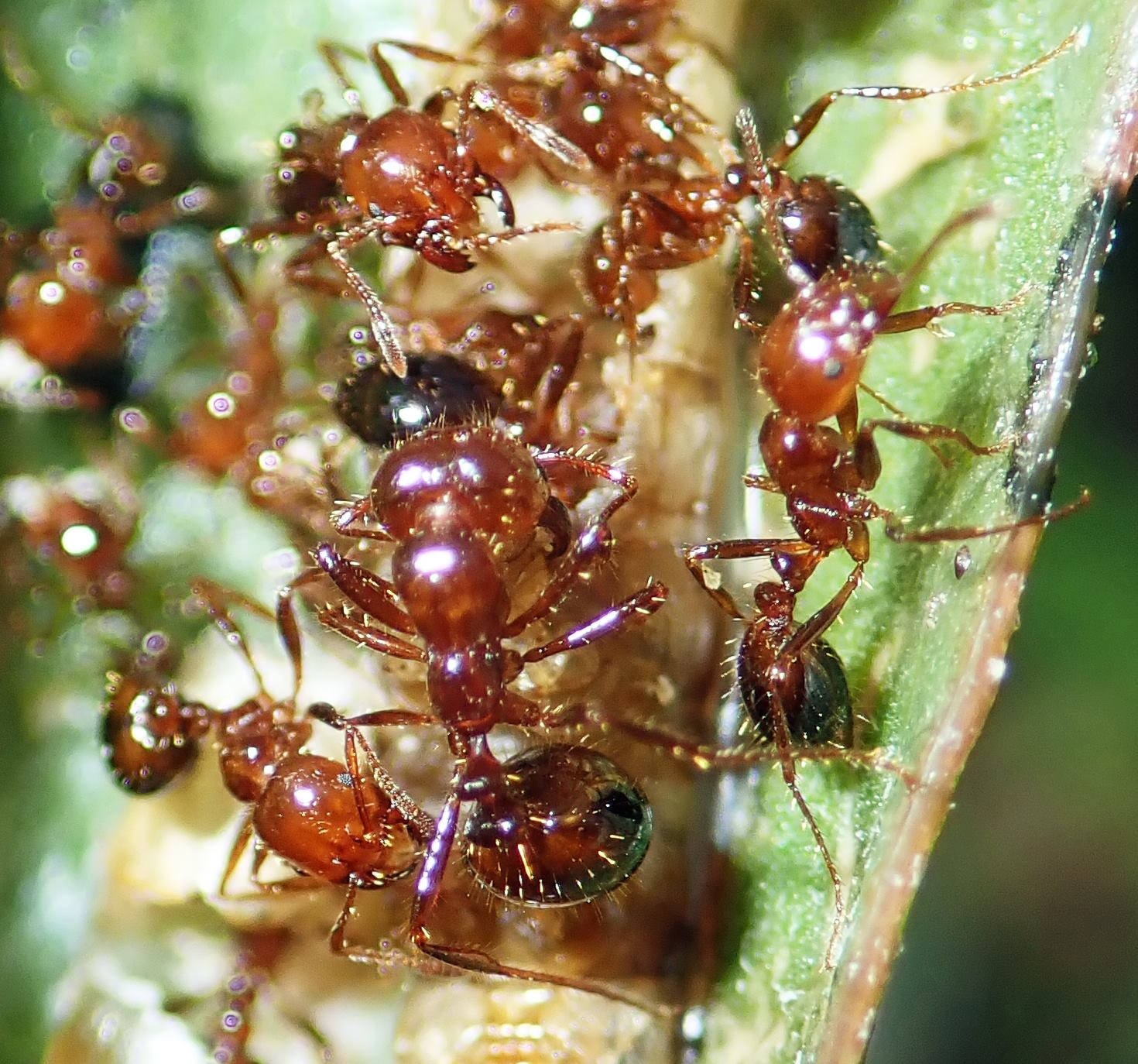This close-up color photograph captures a vivid scene of red ants swarming over a green leaf. The detailed focus reveals one prominent ant in the center, showcasing its three-part body with a shiny reddish-brown hue, complemented by a darker, almost black abdomen. Surrounding this central figure, several other ants can be identified, with four distinctly visible and several more blurred in the background, totaling around ten. The ants exhibit intricate features such as tiny hairs on their thin legs, antennae, and small pincers on their faces, along with a visible eye on one of the ants. They are devouring an unidentifiable, tannish substance partially blurred in the foreground. The image also reflects a shiny texture on the ants, likely from light reflection. The leaf's edges transition into a blurry green, emphasizing the central ant and creating a sense of depth. The nature of the leaf remains indistinct, though it resembles an aloe vera or similar plant, reinforcing the organic, natural setting of this intriguing close-up shot.